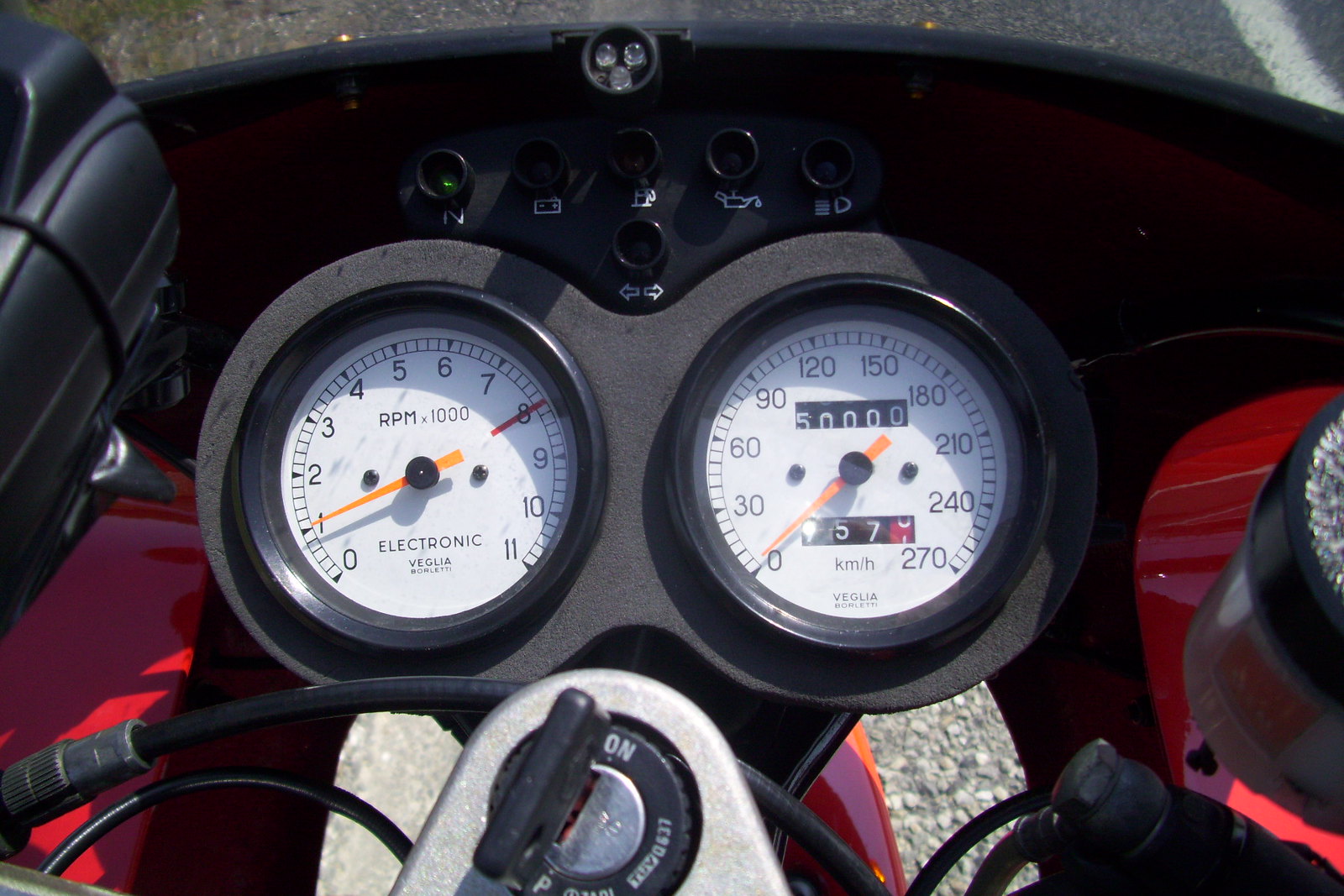This image captures a close-up view of an RPM gauge and a speedometer, likely mounted on a vehicle dashboard. The RPM gauge, positioned on the left, displays a reading of 1,000 RPMs. It has a scale that ranges from 1 (x1000) to 11 (x1000) RPMs. On the right, the speedometer is indicating zero miles per hour. This speedometer's scale maxes out at 270 kilometers per hour. Just below the primary speedometer reading, there is a trip meter showing 157.1 kilometers.

The speedometer also includes a secondary metric at the top, indicating a max speed of 50,000 kilometers per hour, which appears to be part of the design illustration. Below these gauges, a key is visible along with what appears to be an ignition switch. The faces of both gauges are white with black numerals and markings, making the readings clear and easy to interpret. Surrounding the gauges, there's a blend of red and black hues, though the exact elements are indistinguishable in this part of the image. Overall, the image offers a detailed view of the vehicle's instrument panel, highlighting the precise measurements of the gauges.